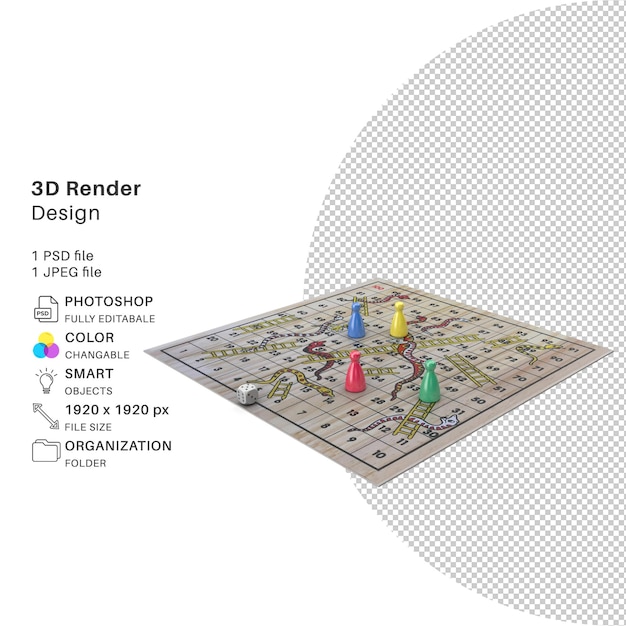The image is a detailed 3D rendered design featuring a game board reminiscent of Chutes and Ladders or Snakes and Ladders, with blue, yellow, red, and green game pieces and a single die positioned on the board. The board appears to float horizontally in space like a magic carpet. The background is primarily white, with a 2D semicircle on the right composed of dotted white and gray lines forming a checkerboard pattern.

On the left side of the image, there is descriptive text and several icons. It says "3D Render Design," and indicates the availability of one PSD file and one JPEG file. The text mentions that the PSD file is fully editable in Photoshop and color changeable, which is emphasized by an icon with three overlapping circles in blue, yellow, and purple. There is also a light bulb icon labeled "Smart Objects." Additionally, the image specifies the file size as 1920x1920 pixels, and there is an icon resembling a sizing arrow indicating adjustable dimensions. Lastly, there is a folder icon labeled "Organization Folder."